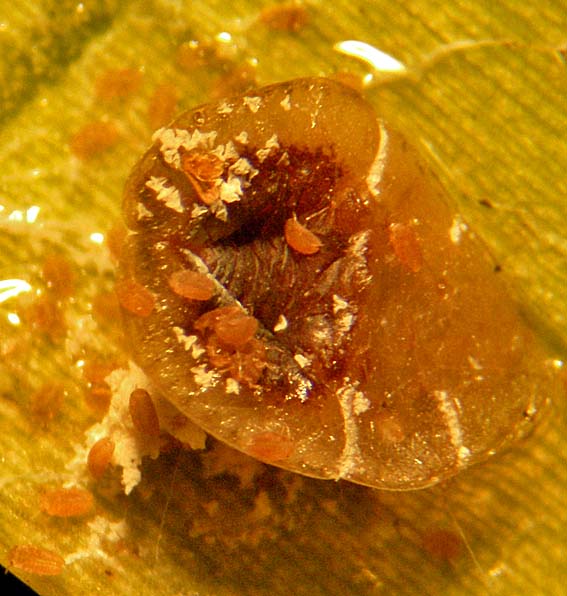The vertical rectangular image depicts a dark yellow, glassy bowl resting on a matching, clear glass plate. The bowl, which appears to have a design incorporating golden hues and white lines, has a peculiar, almost resin-like texture. Upon closer inspection, the dark and orange areas around the bowl feature tiny, orange, bean-sized insects. These insects are scattered both inside and around the bowl, their legs vaguely visible but without discernible eyes. The glass plate beneath the bowl mirrors the bowl's design and rests on a white cloth, possibly a tablecloth. The scene has a peculiar and potentially unsettling quality, evoking images of food, yet the overlay of insect-like entities contributes to its disturbing aesthetic.